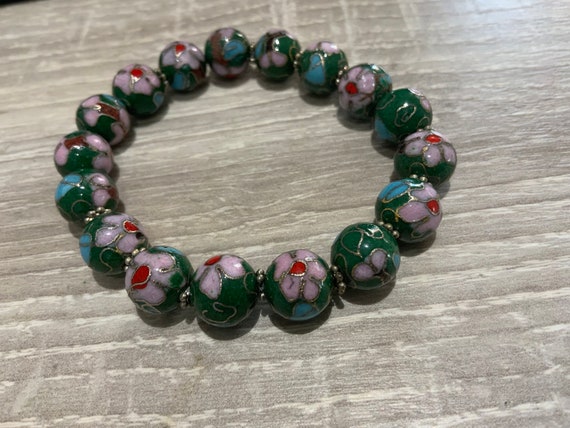This photograph captures a meticulously designed choker necklace, composed of 17 perfectly round, shiny beads arranged in a tight circle to fit snugly around the neck. Each bead features a unique decoration of five-petal flowers, predominantly green with varying placements. At the core of each flower, a small red dot is encircled by a silver ring, adding a vibrant touch against the green background. The necklace is displayed on a surface that appears to be a grey mat with white stripes, adding a contrasting backdrop to the intricately designed beads.